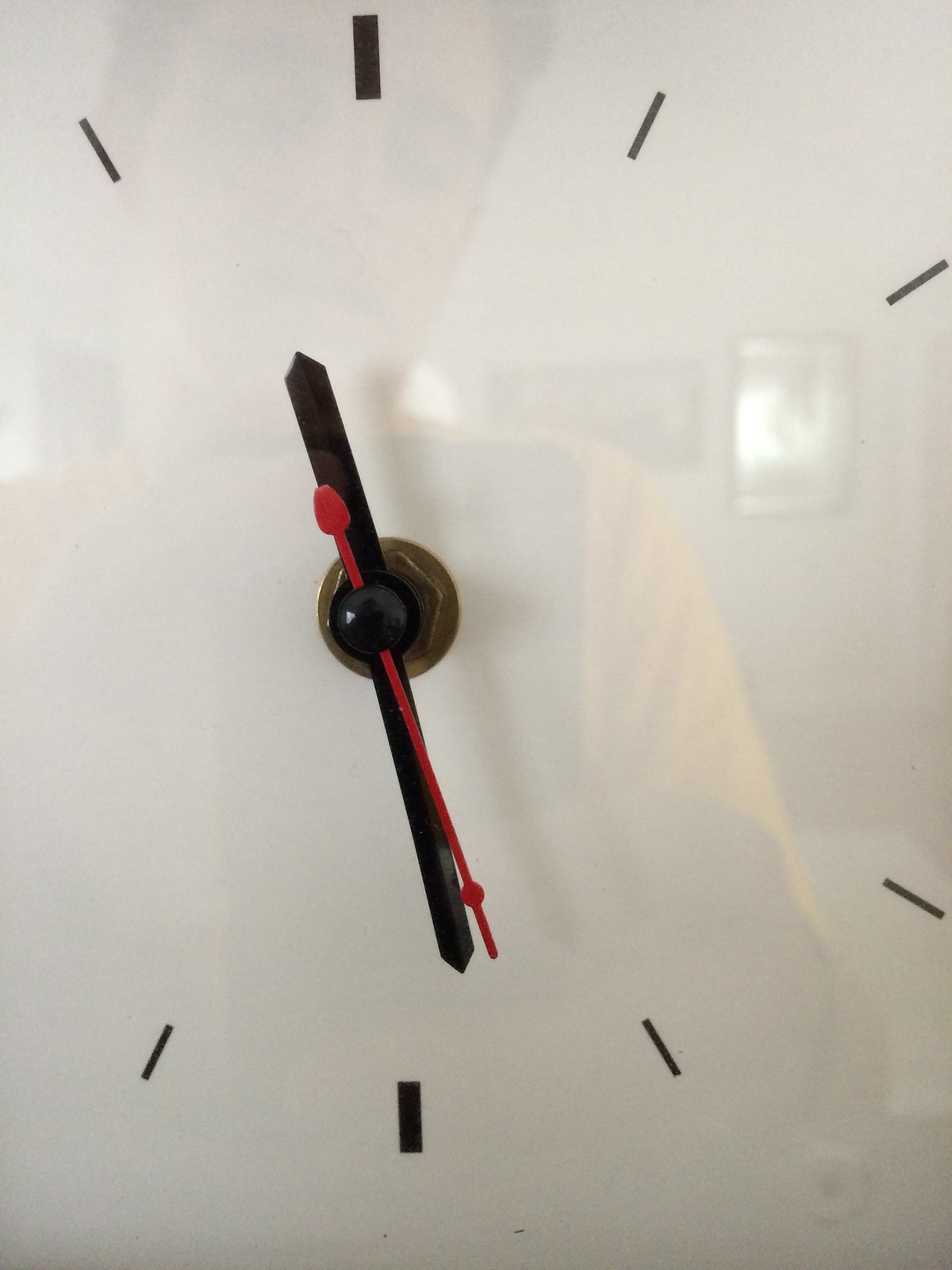This detailed, close-up image captures the partial view of a shiny white clock, showcasing its minimalist design with prominent, thicker lines at the 12 and 6 positions, and thinner lines where the other numbers should be. The clock hands, including a red second hand, are closely aligned, indicating a time of approximately 5:29. Reflecting on the glossy surface of the clock, there's a clear image of a person taking the photo. The individual, a young man wearing a vibrant yellow shirt, holds up his phone to capture the shot. His head is slightly tilted, revealing short, brownish hair. Behind him, the background hints at a room decorated with various pictures on the wall. The overall composition is dominated by the close-up of the clock, creating an intriguing blend of timepiece details and reflective portraiture.